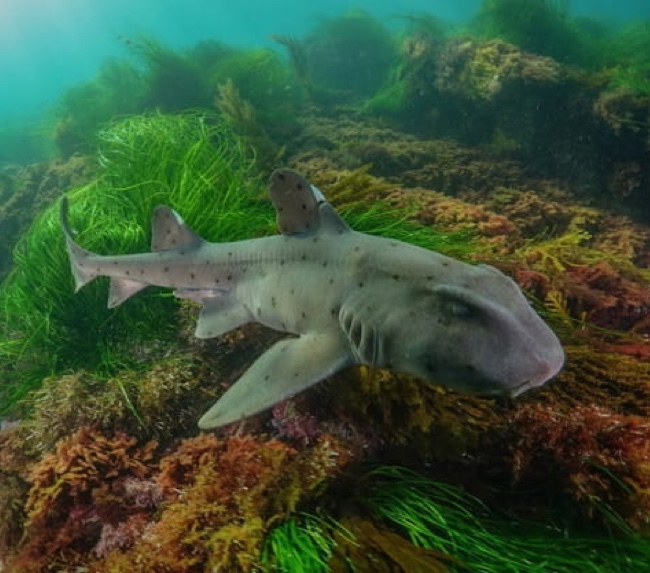A captivating underwater photograph features a shark, likely a leopard shark, swimming gracefully near the ocean floor. The shark, light gray in color, is adorned with scattered black polka dots across its body. Its head is wide and flat, resembling more of a reptile's shape than a typical shark, with large, oval eyes visible on its right side. Each of its top two dorsal fins has a small white splotch, breaking the uniformity of its gray hue. The shark is captured swimming from left to right, its mouth closed and gills clearly visible. Beneath and behind the shark, a vibrant coral reef showcases striking orange and yellow hues, interspersed with clumps of bright green grass, resembling algae. The murky, turquoise water adds a dreamy, hazy effect to the image, accentuating the serene beauty of this underwater scene.